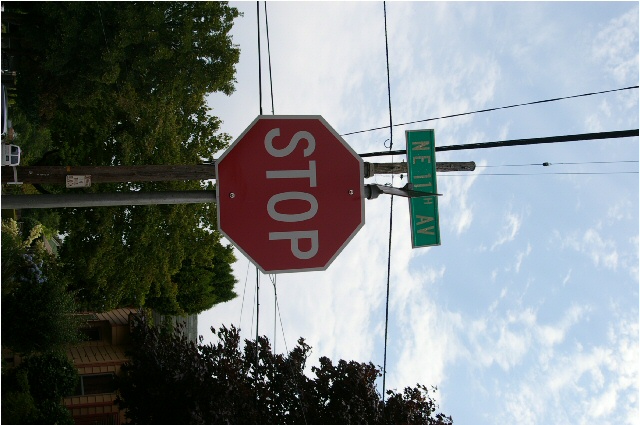This image, captured outdoors, is a photograph that has been rotated 90 degrees clockwise. To view it in the correct orientation, one must turn their head accordingly. The scene depicts a blue sky with the sun positioned low, suggesting either sunrise or sunset. Central to the composition is a classic red stop sign mounted on a metal post. Directly above the stop sign, there is a green street sign with white text that reads "North East 11th Avenue." In the background, electrical pylons crisscross the sky. The surrounding environment features numerous tall, green trees, indicating a verdant, tree-lined street.